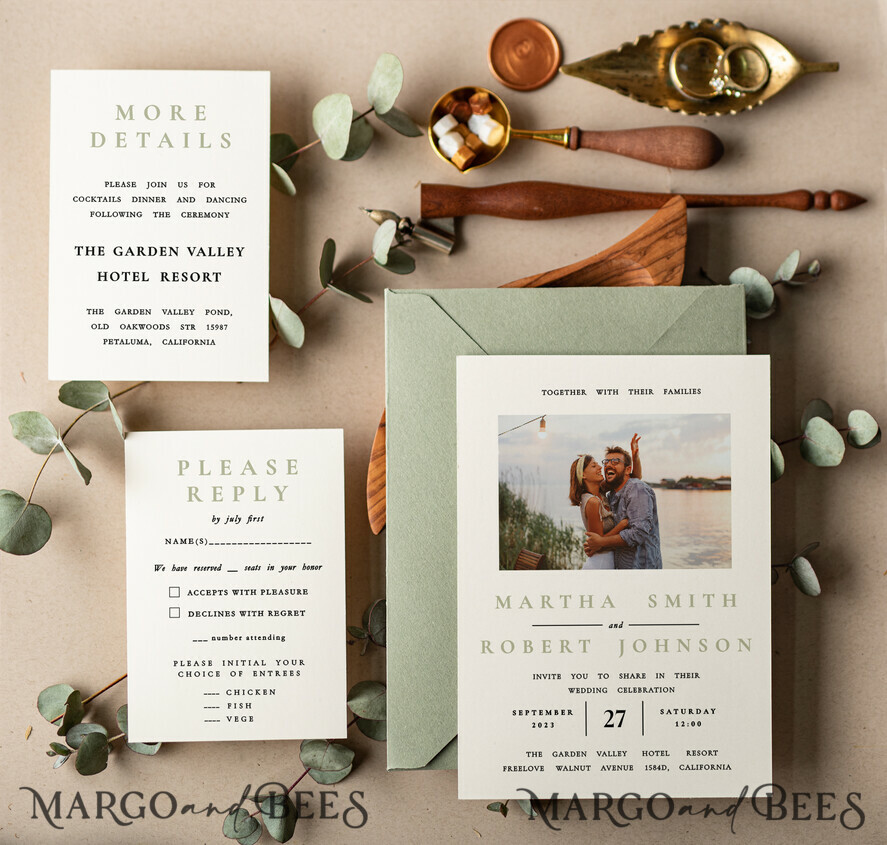The image showcases a series of elegantly designed wedding stationery items, all branded by Margot and Bees, arranged artistically amidst eucalyptus leaves and various decorative objects. The main focus is on a white wedding invitation, featuring light green and black lettering, which displays a joyful picture of Martha Smith and Robert Johnson hugging and smiling. The text on the invitation reads, "Together with their families, Martha Smith and Robert Johnson invite you to share in their wedding celebration, September 27th, 2023, Saturday, 12 o'clock, at the Garden Valley Hotel Resort, Free Love, Walnut Avenue, California."

To the left of the invitation, there's an RSVP card in matching colors—mint green, white, and black—stating, "Please reply by July 1st," with spaces to fill in guest names, indicate the number of guests, accept or decline the invitation, and select meal preferences from options such as chicken, fish, and vegetarian. Above this is another card with the same color scheme offering additional details, reading, "More details: please join us for cocktails, dinner, and dancing following the ceremony, at the Garden Valley Hotel Resort, the Garden Valley Pond, Old Oakwoods, Petaluma, California."

All of this stationery is garnished with a delicate touch of nature, reinforced by the surrounding eucalyptus leaves and earthy, brown figurines. The bottom of the photo prominently features the branding, "Margot and Bees," emphasizing the company's focus on natural-themed wedding invitations.